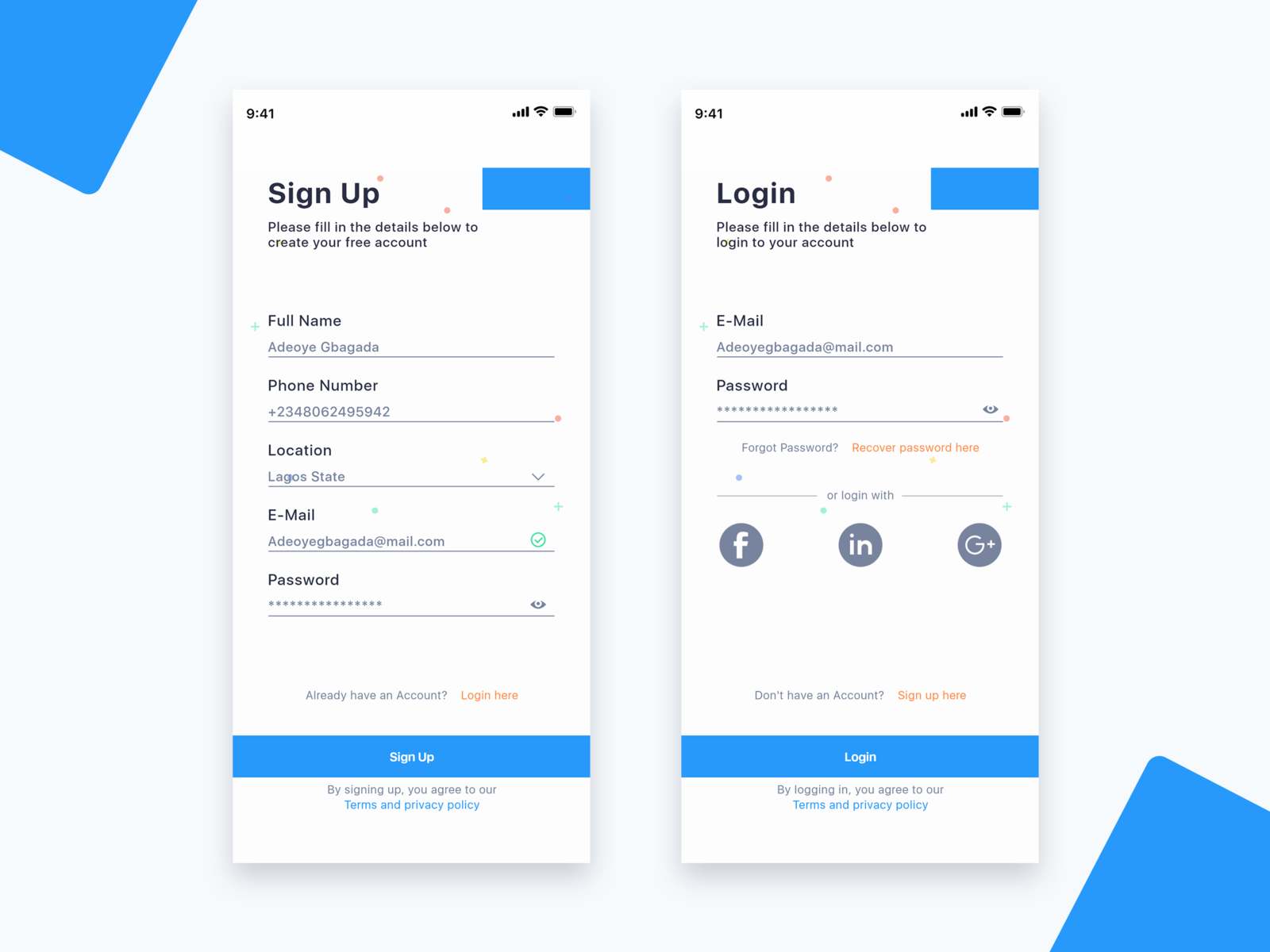This image displays a composite screenshot set against a solid white background, adorned with two blue geometric shapes located at the upper left and lower right corners. The main feature includes two cell phone-sized screenshots embedded within the image. 

The prominent screenshot on the right showcases a typical smartphone status bar at the top with the time "9:41" displayed in black text. The status bar also shows fully lit signal bars, an active Wi-Fi icon, and a fully charged battery symbol. Below this, the screen displays a login prompt against a white background, with the text, "Please fill in the details below to login to your account" in black font.

The login interface includes a text field labeled "Email," pre-filled with "adoebgota@mail.com." Directly below this is a password field, awaiting user input. At the bottom of this screenshot, there are two recognizable social media icons for Facebook and Google+, suggesting alternative login options.